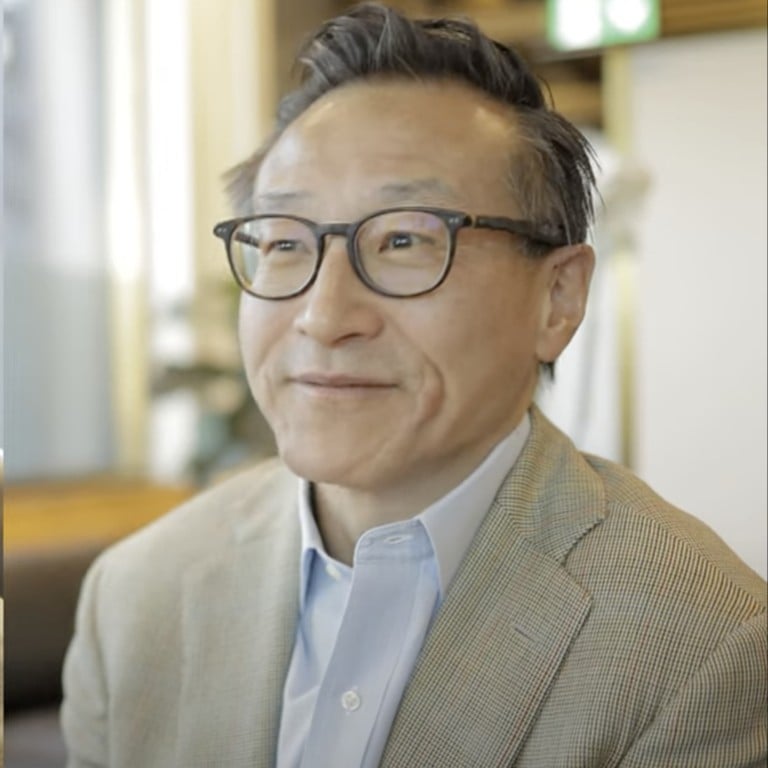The photograph features an older Asian man with a mix of graying and black, slightly messy hair. He has dark brown eyes framed by dark brown or black glasses, and his face exhibits light wrinkles. The gentleman appears to be well-dressed in a light blue button-up shirt with the top button undone, underneath a brown jacket adorned with a faint plaid pattern. He holds a subtle smile as he looks slightly away from the camera, sitting still for the portrait. The background is a blurred indoor setting with indistinct colors, focusing the attention fully on him.